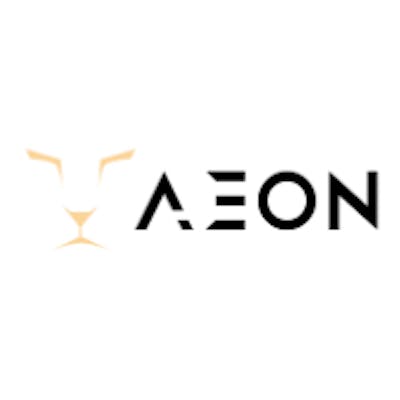The image features the text "Aeon" in a bold, abstract black font, with portions of the A and E slightly obscured, lending a unique, innovative flair. Set against a predominantly black and white background, the centerpiece is an abstract logo reminiscent of a lion or tiger's face, with discernible eyes, nose, and part of the mouth peering out from the left side. The composition is slick and professional, evoking the aesthetic of high-end branding, akin to luxury car advertisements such as those from Audi. The overall design is straightforward and aims to capture attention through its minimalistic yet striking visual appeal.